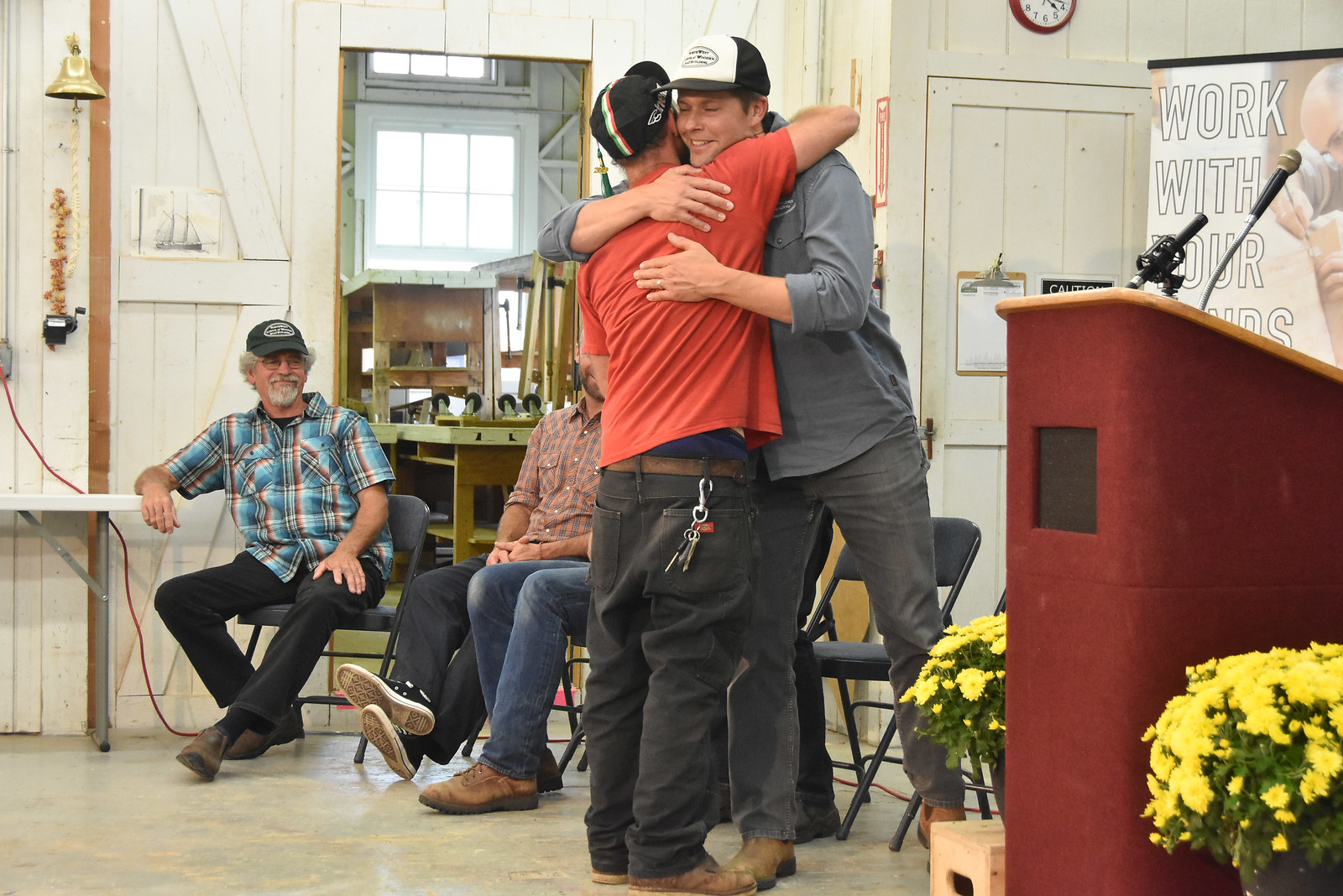This photograph captures a heartfelt moment between two men embracing in an indoor setting that resembles a workshop or informal meeting space. The man facing away from the camera wears an orange T-shirt, black jeans, and brown shoes. A key hook is attached to his belt loop. The man he is hugging sports a gray shirt with rolled-up sleeves, black jeans, and brown shoes. Both men are wearing baseball caps.

In the background, two other men are seated on folding chairs, smiling warmly as they observe the embrace. To the right of the hugging pair stands a red podium adorned with a microphone and flanked by yellow flower arrangements. Behind the podium, a partially visible sign reads, "work with your..," suggesting an event or workshop, possibly centered around teamwork or father-son activities. The overall atmosphere in the image appears positive and supportive.